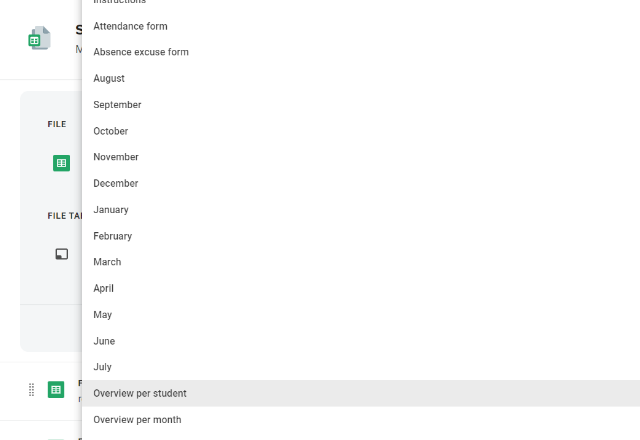Screenshot of a detailed list, displayed in a white box with various forms and month names. The list includes options such as "Attendance Form" and "Absence Excuse Form." Below these, the months from "August" to "July" are sequentially listed. Additionally, two specific views are presented: "Overview per Student," which is highlighted in gray, and "Overview per Month." The layout suggests an organized system for tracking and managing student attendance and absences throughout the academic year.